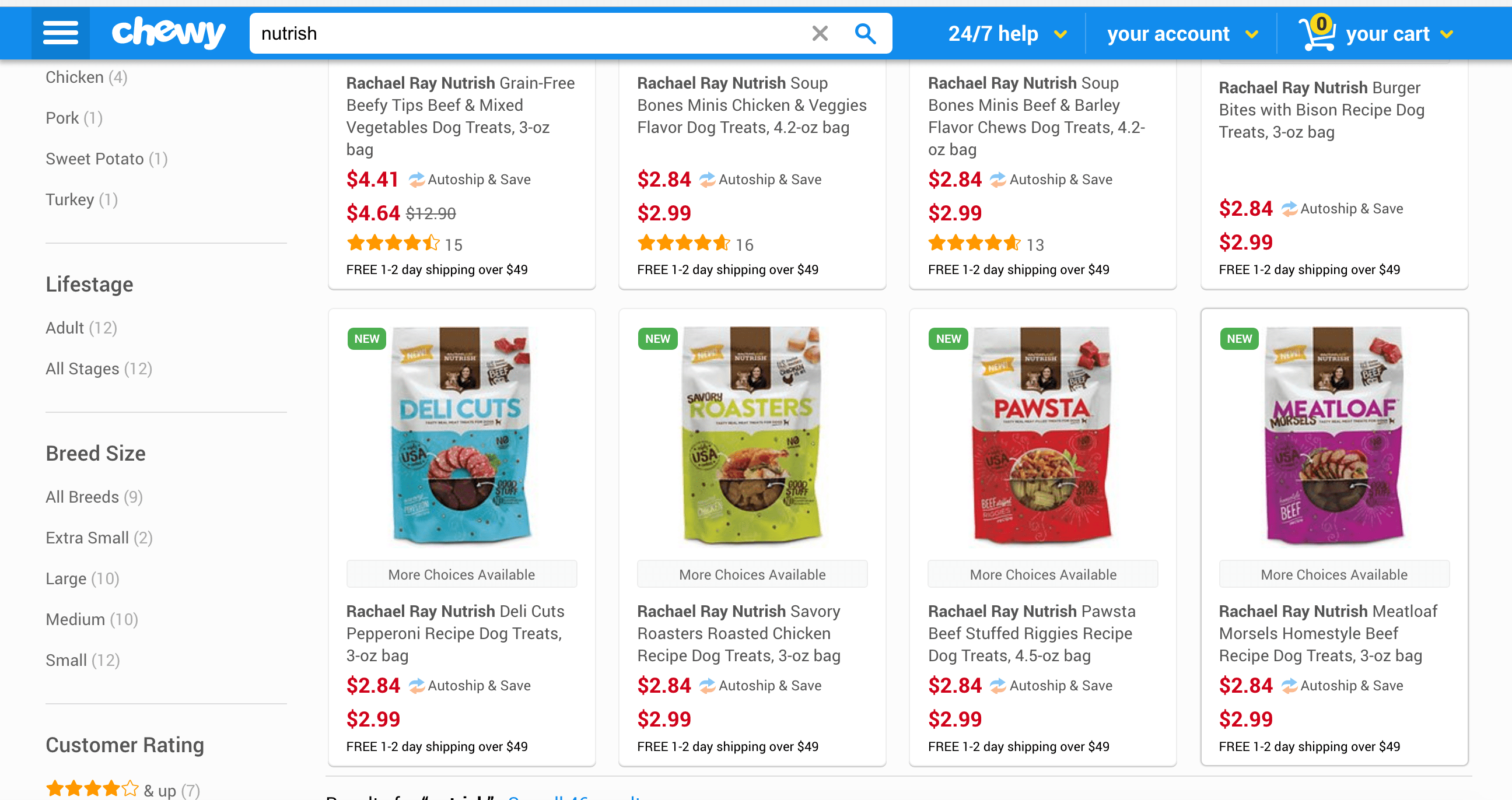The image depicts a webpage from Chewy, an online pet retailer. At the top left corner, there's the Chewy logo, accompanied by a navigational bar that includes a search box pre-filled with the word "Nutrish," an 'X' button, and a magnifying glass icon. To the right, options for 24/7 help and your account, both indicated with downward arrows, are present. The top navigation also features a shopping cart icon.

On the left side of the page, there is a detailed filtering menu with several categories:
- Protein options: Chicken (1), Pork (1), Sweet Potato (1), Turkey (1)
- Life stages: Adult (12), All stages (12)
- Breed sizes: All breeds (9), Extra small (12), Large (10), Medium (10), Small (12)
- Customer rating: 4 stars and up

The main content area showcases products under the "Rachael Ray Nutrish" line of dog treats. There are several bags with distinct colors and labels:
- A blue bag labeled "Deli Cuts"
- A green bag
- A red bag labeled "Paw"
- A purple bag labeled "Meatloaf"

Each bag prominently displays the "Rachael Ray Nutrish" branding, along with their respective prices and a note indicating free one to two-day shipping on orders over $49.

Above these visible product listings, there are mentions of four additional product listings, also under the Rachael Ray Nutrish brand, displaying related pricing and shipping information, though the images for these products are not shown.